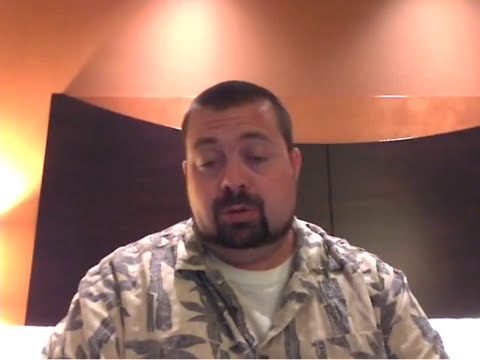The image is a low-quality, slightly blurry color photograph of a Caucasian man sitting on a bed in what appears to be a hotel room, characterized by its brightly lit, plain background. The man, who is a bit overweight, sports a crew cut hairstyle and has a thin beard outlining his jawline, complemented by a goatee. He is wearing a white undershirt beneath a tan and gray button-down shirt adorned with palm tree and floral patterns. His serious demeanor, with eyebrows and eyelashes turned down and a pursed mouth, gives the impression that he is either speaking or about to speak. Behind the man is a curved brown wooden headboard, and the room features various light sources, including a yellow glow from the left and a rich orange hue reflecting off the ceiling.